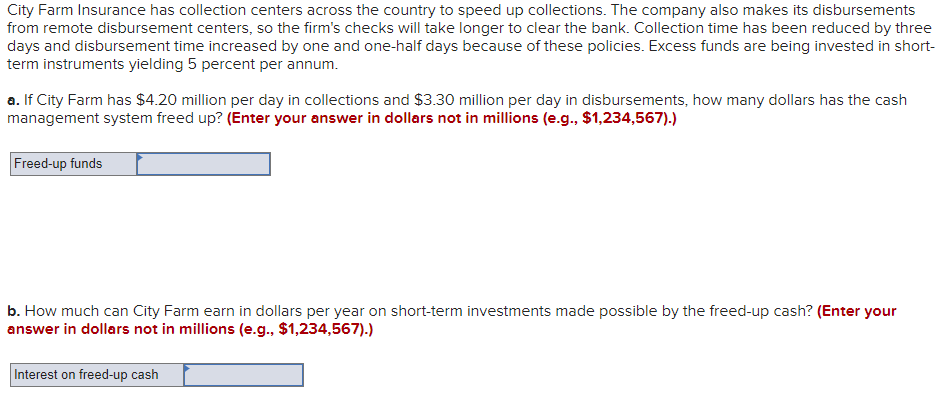This is an image of a worded math problem, possibly from a textbook or journal, displayed on a plain white background. The problem discusses City Farm Insurance, which has collection centers across the country to expedite collections and remote disbursement centers to delay check clearance. This strategy reduces collection time by three days and increases disbursement time by one and a half days. Excess funds are invested in short-term instruments yielding 5% per annum. The problem is divided into two parts: 

A. If City Farm collects $4.20 million per day and disburses $3.30 million per day, determine the amount of funds that the cash management system has freed up. Instructions note to enter the answer in dollars, not millions, with an example format provided.

B. Calculate the annual earnings in dollars from the short-term investments made possible by the freed-up cash, with a space to enter the answer in dollars, not millions, following the provided format.